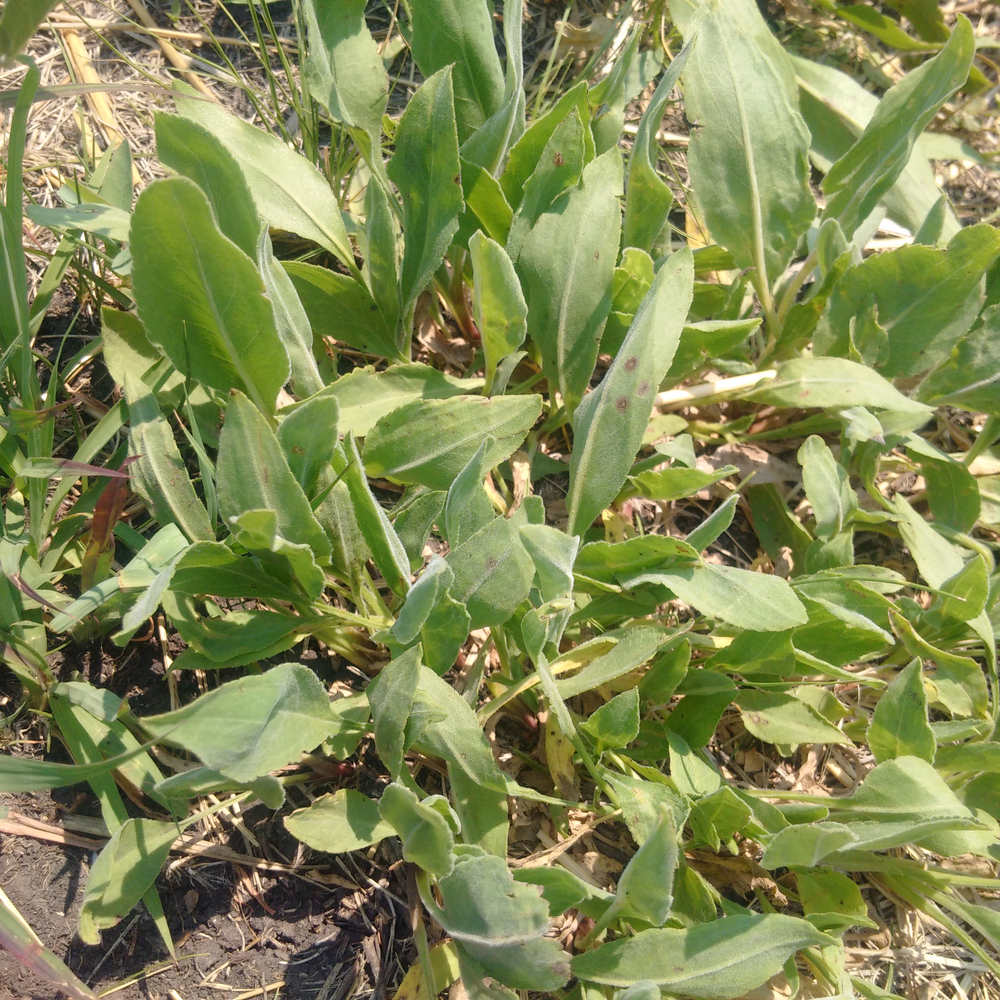This image features a bright outdoor scene abundant with vegetation. Dominating the center are soft, thick, light green leaves, densely clustered across the entire frame. A few of these leaves display brown spots. The ground showcases a mix of yellowish-brown dried grass and darker brown dirt, particularly noticeable in the bottom left corner. Additionally, the bottom left includes a small patch of concrete or asphalt. Scattered throughout are various sticks and twigs, with long dead shoots of what seems to be bamboo or straw in the top left. In the center left, a single long blade of grass rises from the ground. The photograph, taken from a top-down perspective, reveals the sun's rays illuminating the scene, indicating a bright, sunny day during a warm season. The overall color palette includes shades of green, brown, yellow, and gray, reflecting the natural, untamed outdoor setting.